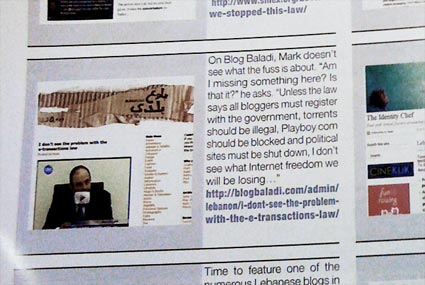The image appears to be a collage, potentially a poster but possibly a screenshot, composed of multiple website screenshots. The bottom left of the image has a bend with a reflection, suggesting it might be a printed poster rather than a digital screenshot. The collage is divided into six squares, but only one is fully visible while the edges of others are partially shown.

The visible section features a screenshot from the website "BlogBaladi," depicting an individual sitting at a desk in a suit. The surrounding text is largely unreadable, but a quote beside the image reads: 

"On BlogBaladi, Mark doesn't see what the fuss is about. He says, 'Am I missing something here? Is that it? Unless the law says all bloggers must register with the government, torrents should be illegal, playboy.com should be blocked and political sites must be shut down, I don't see what internet freedom we will be losing.'"

This quote suggests that the blogger, Mark, disagrees with the notion that internet freedoms are at risk based on the issues he discusses. A link to his blog is also included.

The remaining five sections presumably follow a similar format, with each featuring an image from a site and related commentary, although the text in these sections is not legible in the current view.